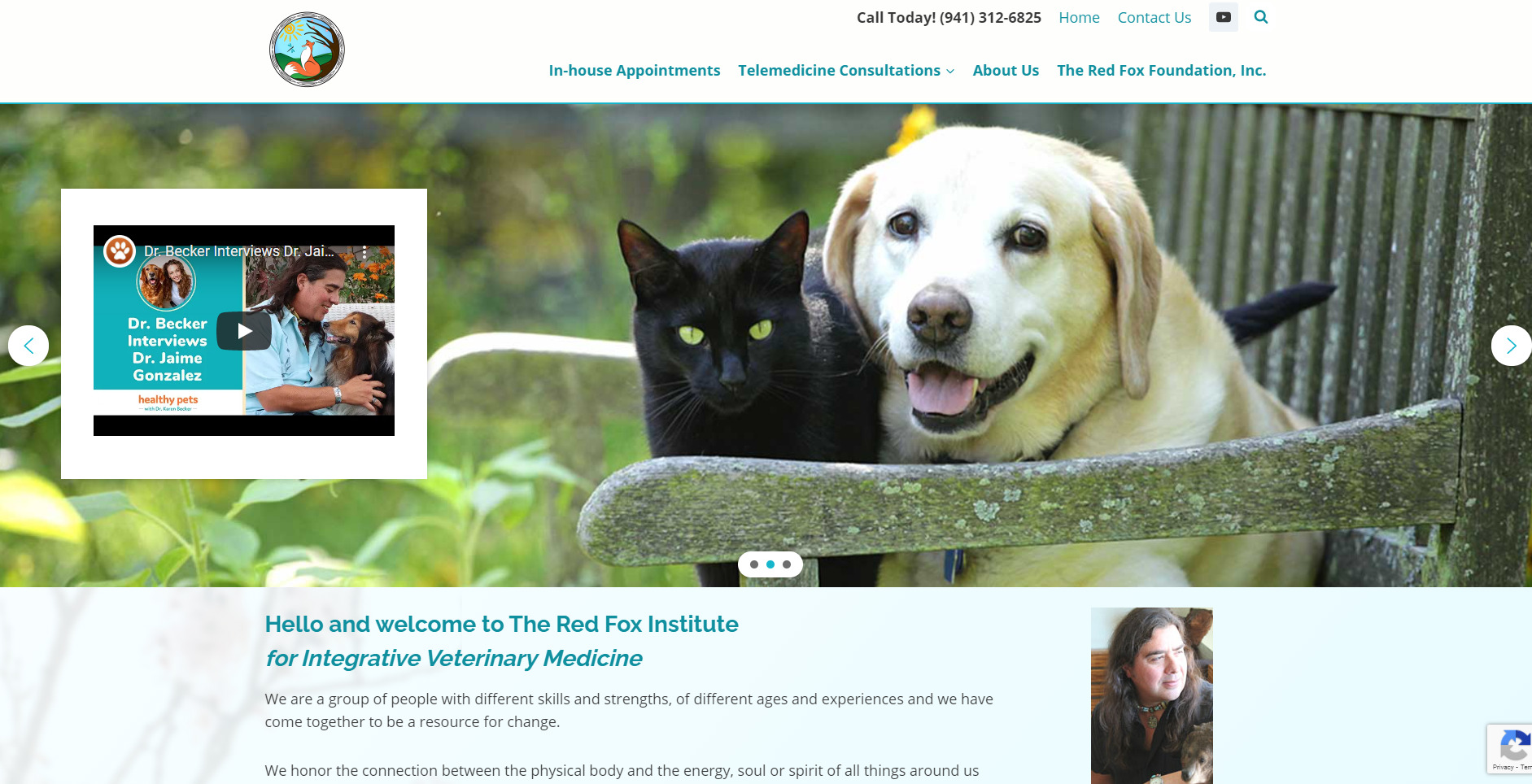Screenshot from a veterinarian website:
--------------------------------------

On the left side of the image, there is a logo featuring a whimsical little fox standing underneath a tree with rays of sunshine partially illuminating the scene. To the right of the logo are two lines of text, the first line reads “Call today 941-312-6825.” Directly below, there are navigation options including "Home" and "Contact Us." Following this, users can also choose from "In-house Appointments," "Telemedicine Consultations," "About Us," and information about "The Red Fox Foundation Inc."

Centered prominently in the middle of the image is a photograph of a dog and a cat sitting together on a chair outdoors, basking in the sunlight. The cat is black with striking green eyes, while the dog has a beige or blonde coat. Adjacent to them is a clickable video which promises further information or entertainment.

Below the photograph, a section of blue text reads, "Hello and welcome to the Red Fox Institute for Integrative Veterinary Medicine." Beneath this headline, smaller black text states, "We are a group of people with different skills and strengths, of different ages and experiences. We have come together to be a resource for change." Further down, it continues with, "We honor the connection between the physical body and the energy, soul, or spirit of all things around us," but the remainder of the text gets cut off.

To the right of this informative block is an image of a man with long hair, holding a small animal, though the details are somewhat indistinct from the description provided.